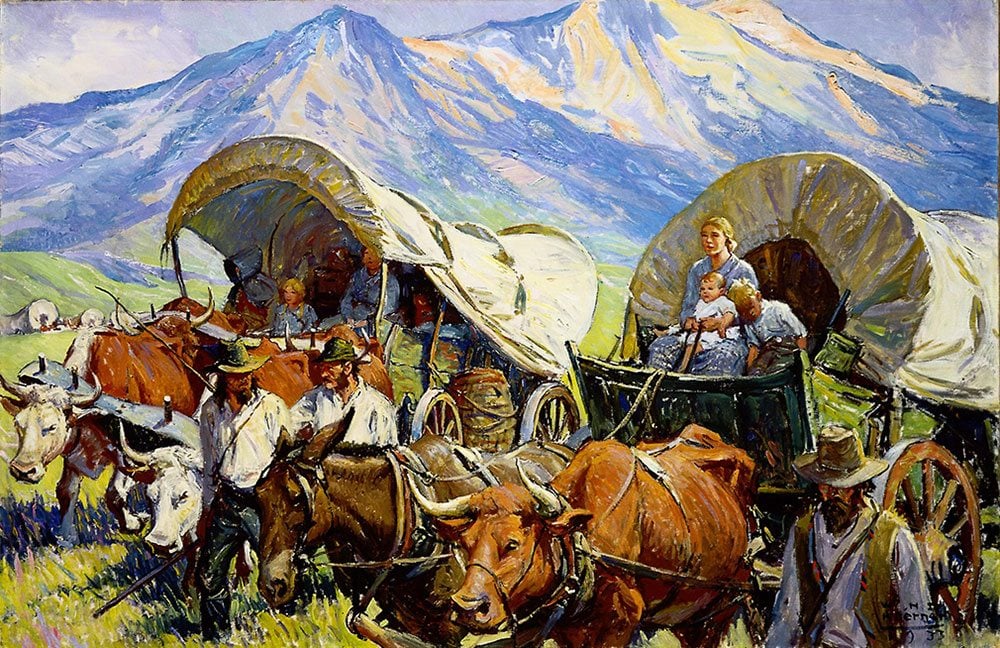This detailed painting captures a vivid scene of settlers journeying westward, likely along the Oregon Trail, towards California or Oregon. The artwork shows two covered wagons, often referred to as caravans, each with their classic white canvas covers. The first wagon, positioned to the right, is pulled by an ox and a horse. A woman dressed in a blue dress sits at the front, holding the reins with a baby on her lap and a young boy, likely preschool-aged and blonde like his mother, who appears to be dozing off beside her. The children wear white outfits, adding to the contrast of the scene.

The second wagon, located on the left, is drawn by two steers and also has a woman managing the reins. Accompanying the wagons are several men walking alongside. One man, situated to the bottom right, sports a beard, wears a white shirt and a vest, and holds a rifle. Other men are similarly dressed in white shirts and hats. The vivid colors in the painting include various tones such as ox reddish-brown, white, tan, beige, green, blue, and blonde, adding richness to the landscape.

In the background, high mountains tower over the scene, emphasizing the challenging journey. The green grass suggests they have reached a fertile area, possibly near the end of their trek. Together, these elements create a detailed portrayal of pioneer life and the arduous journey of settlers on the historic Oregon Trail.